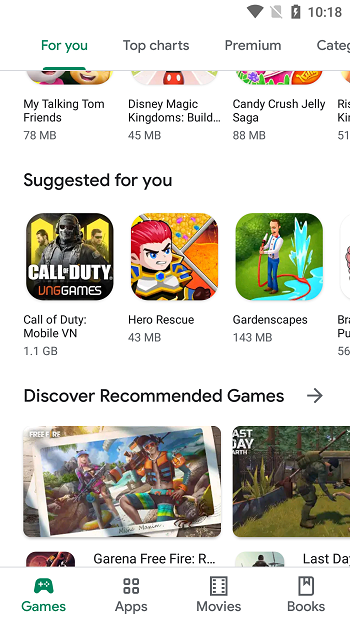The smartphone screen displays a "Games For You" page within an app, likely the Google Play Store. In the top right corner, there is a black battery icon with a white lightning bolt, indicating charging status. The time, "10:18," is displayed in black text nearby. Next to the battery icon, there are several smaller black and gray icons.

Beneath these, we have navigation tabs including "For You," "Top Charts," "Premium," and an unclear tab starting with "CATE." The "For You" tab is highlighted in green, indicating it is the active section.

At the bottom of the screen, there are more navigation options: "Games," "Apps," "Movies," and "Books." The "Games" tab is highlighted in green as well, indicating the user is currently browsing games.

The main portion of the screen showcases the section titled "Suggested For You" in black text. Below this header, three game options are displayed in squares with rounded corners: "Call of Duty," "Hero Rescue," and "Gardenscapes."

Further down, another header in black text reads "Discover Recommended Games," followed by a forward arrow icon. Below this, we see a box featuring "Garena Free Fire," alongside another partially visible game title "Last Day," though only the letters "DNA" are fully readable.